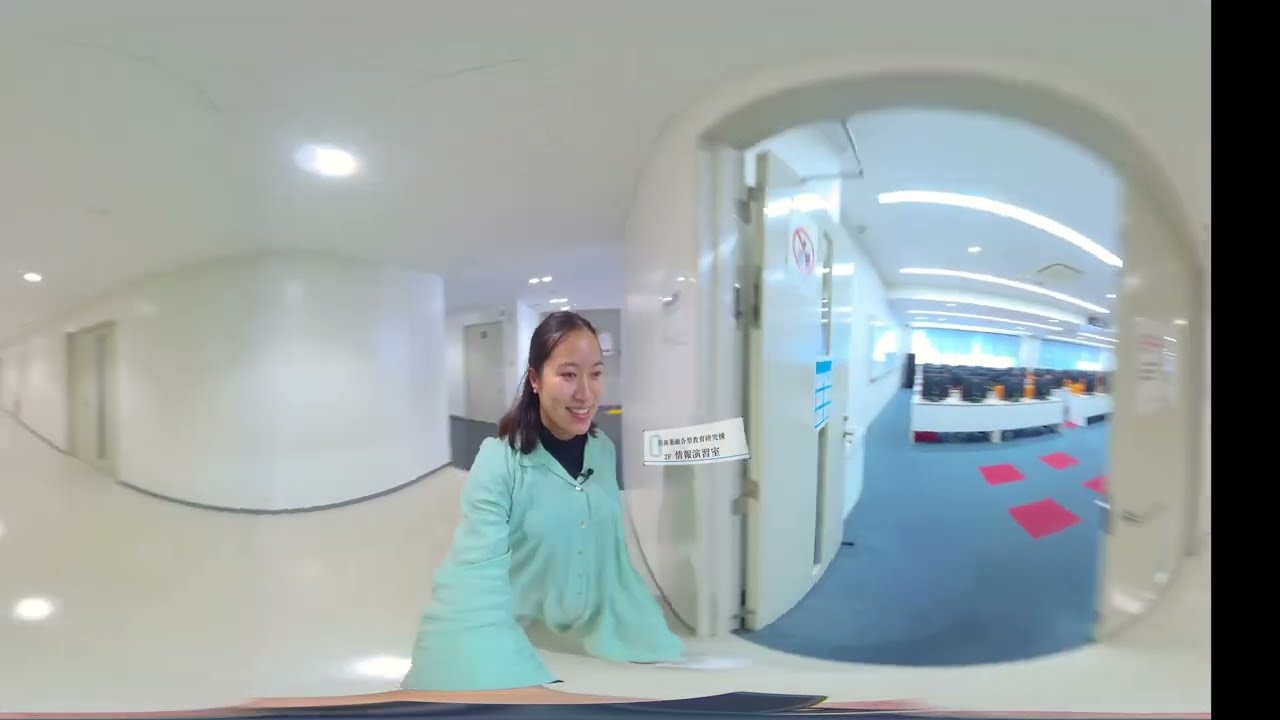The image is a fisheye view of an Asian woman with black hair, possibly of Chinese descent, standing in the midst of a large, predominantly white room. She is wearing a green jacket with a hood and buttons, layered over a black shirt. A small microphone is clipped to her collar, suggesting she might be presenting. Behind her, the room features rows of white tables topped with numerous computer monitors, illuminated by fluorescent lights. The floor is covered in a gray carpet with four distinct red squares. Multiple white walls and doors add to the room's sterile appearance, giving the impression of a hospital, university, or tech company. Nearby, a door is open with a sign bearing Chinese characters and a warning label. The overall ambience of the room is clinical and bright, with white puck lights dotting the ceiling.